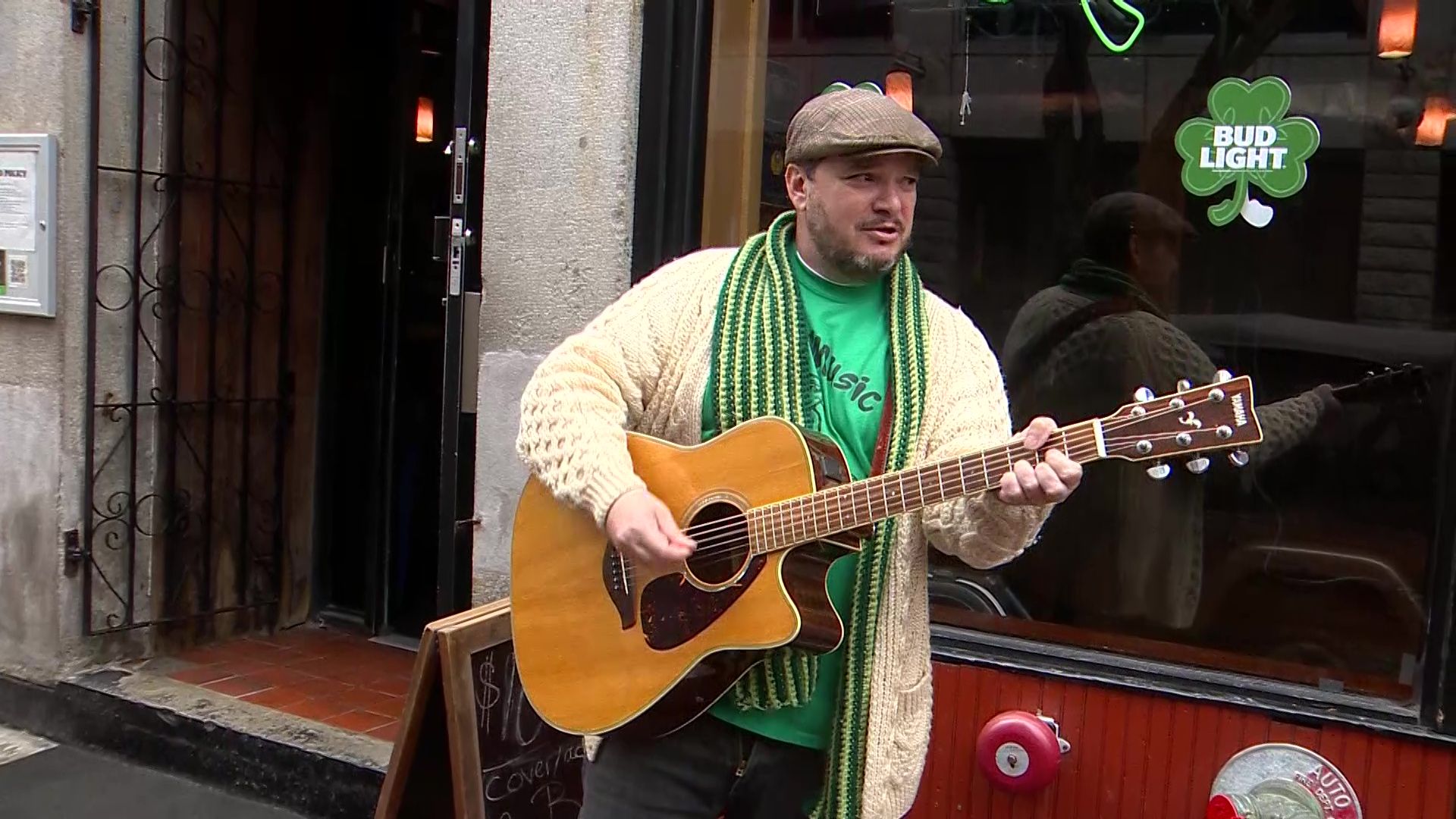In this close-up photograph, a street performer is captured in front of an establishment, likely a restaurant, due to the visible Bud Light logo on a green shamrock sticker affixed to the large window behind him. The performer is standing on the sidewalk, playing a guitar in motion while looking to his left. He is dressed in a quilted jacket with a white sweater, layered over a green t-shirt and an underlayer that appears white. A green and yellow knitted scarf with stripes wraps around his neck, complementing his brown newsboy cap. The guitar he holds features a light brown, yellowish bass with a dark brown neck. On the left side of the image, there's a door entrance to the shop with black iron bar gates, and part of a sideboard is visible at the corner near the sidewalk. The scene is brightly lit, suggesting it is daytime.